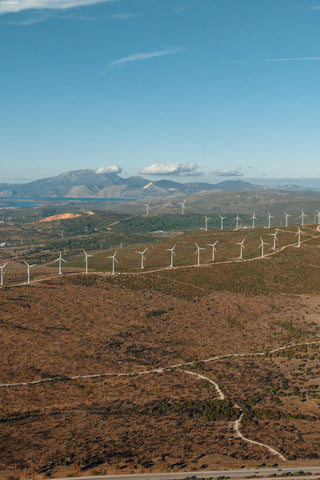This image is an aerial color photograph displaying a sprawling wind farm set in a desert-like landscape. The vantage point of the photo seems to be from a high altitude, possibly from an aircraft, given that the scene includes bright white puffy clouds hovering at the level of distant mountains, which border the furthest section of the image. The sky above is a vibrant blue, contrasting with the earthy tones below.

Beneath the clouds and mountains, the terrain spreads out in a patchwork of varying shades of brown, light red, and dark brown, broken by occasional bodies of serene blue water. The foreground of the image reveals a scrubby, flat expanse of brown land, dotted with patches of green vegetation. Dirt roads cut through this landscape, with one prominently zigzagging from the lower right and joining another that runs horizontally.

Cutting a conspicuous line across a ridge in the middle of the photograph, approximately 20 or more white wind turbines sit, each equipped with three blades. These turbines extend across the horizon, some nestled into greener hills in the near distance, while others are scattered upon the ridge and beyond. Another dirt road meanders alongside these wind turbines, curving off to the right before descending back down to the left.

In the far distance, a body of water lies to the left, with a mountain range rising majestically behind it. This photograph captures an intriguing mix of natural beauty and human intervention, illustrating the scale of wind power infrastructure amidst a diverse and colorful landscape.